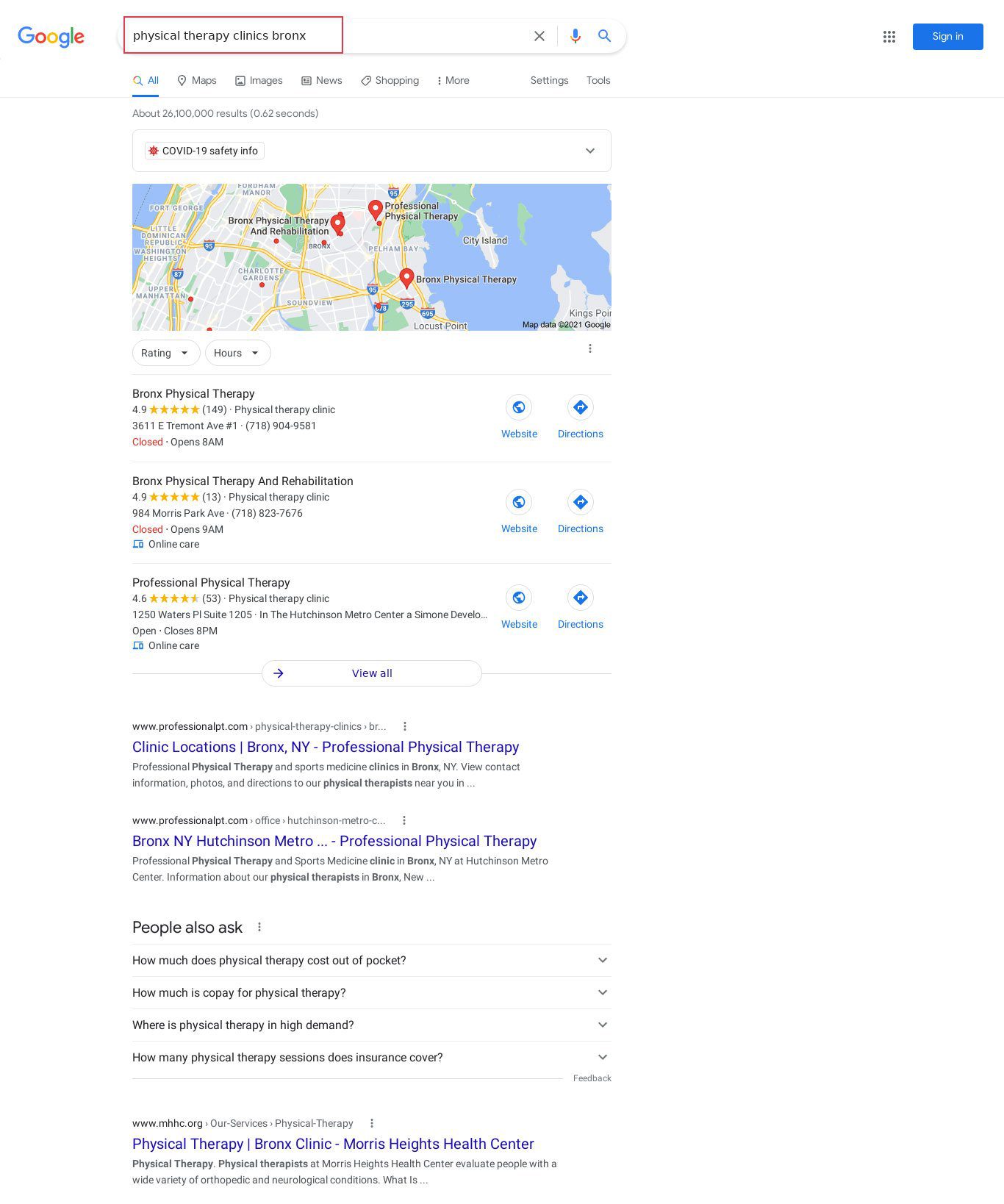The image depicts a Google search results page with a pristine white background. Dominating the top is the iconic Google logo, displayed in its familiar blue, red, yellow, and green lettering. To the right of the logo, the search query "Physical Therapy Clinics Bronx" is prominently highlighted within a red box. Adjacent to the query are three icons: an 'X' for clearing the search bar, a microphone for voice search, and a magnifying glass for initiating a search. Further to the right, a blue "Sign In" button is visible.

Directly beneath the search bar, the standard Google search options are listed: All, Maps, Images, News, Shopping, More, Settings, and Tools, with "All" being selected. Below this navigation bar, the search results indicate approximately 26,100,000 results found in 0.62 seconds.

The first result shows a notice about COVID-19 Safety Information followed by an embedded Google Maps snippet highlighting the Bronx area. Just below the map, there is a section labeled "Ratings and Hours." Following this, there are clickable links to various physical therapy facilities: "Bronx Physical Therapy," "Bronx Physical Therapy and Rehabilitation," and "Professional Physical Therapy," each offering options for directions or visiting the website. An option to "View All" links is provided underneath these listings.

Below this, the search results list various webpages related to physical therapy clinics in the Bronx, such as the "Bronx New York Professional Physical Therapy," and "Bronx New York Hutchinson Metro Professional Physical Therapy." Further down, the "People Also Ask" section presents drop-down questions like "How much does physical therapy cost out-of-pocket?" and "How many physical therapy sessions does insurance cover?"

Finally, another webpage link for the "Physical Therapy Bronx Clinic" is listed towards the bottom, providing additional information on available services.